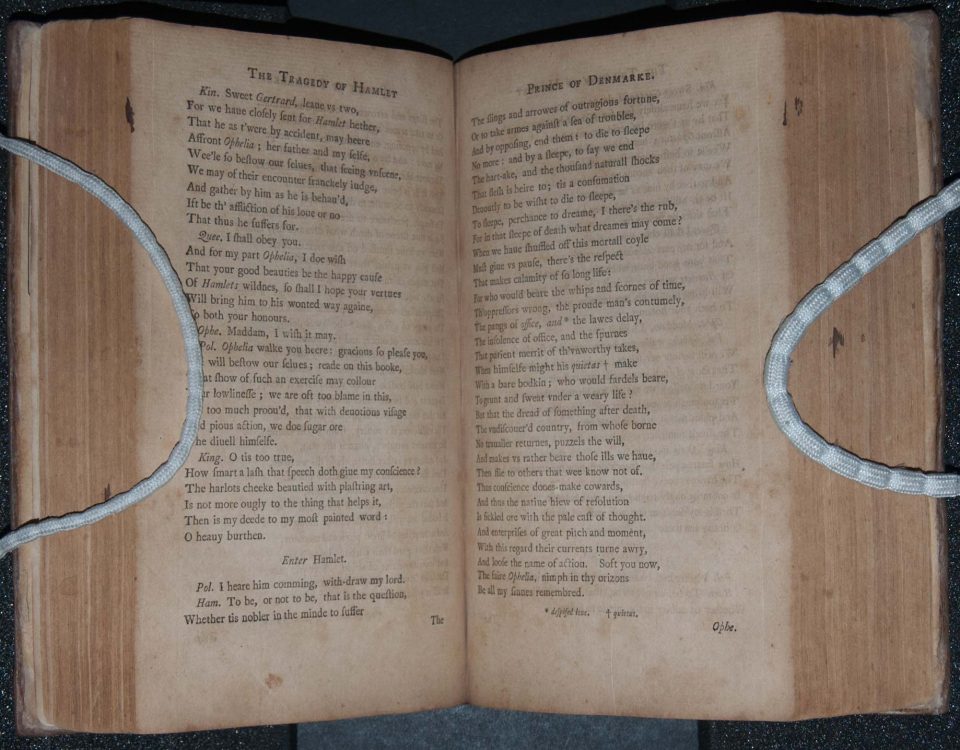The image is a color photograph of a very old, open book, likely from the early 1900s, laid out so that both the left and right pages are visible. The book appears to be weathered, with pages that are thin enough to let the text on the opposite side somewhat show through. The pages are a brownish-beige or yellowish-white color, consistent with significant aging and adorned with visible stains.

The title at the top of the left page reads "The Tragedy of Hamlet," while the right page's title reads "Prince of Denmark," indicating that this is a text from Shakespeare's famous play, Hamlet. The text on the pages is black, with a significant block of text situated below the titles.

Additionally, two synthetic ropes, white with hints of gray, are draped over the book—one over the left page and another over the right—each forming loops that extend off the sides of the image, appearing as hooks or loops resting in front of the pages. The background of the image is empty, save for a hint of blue coloring that adds no discernible detail. The overall condition and appearance of the book imply that it contains hundreds of pages and is opened approximately to its middle.